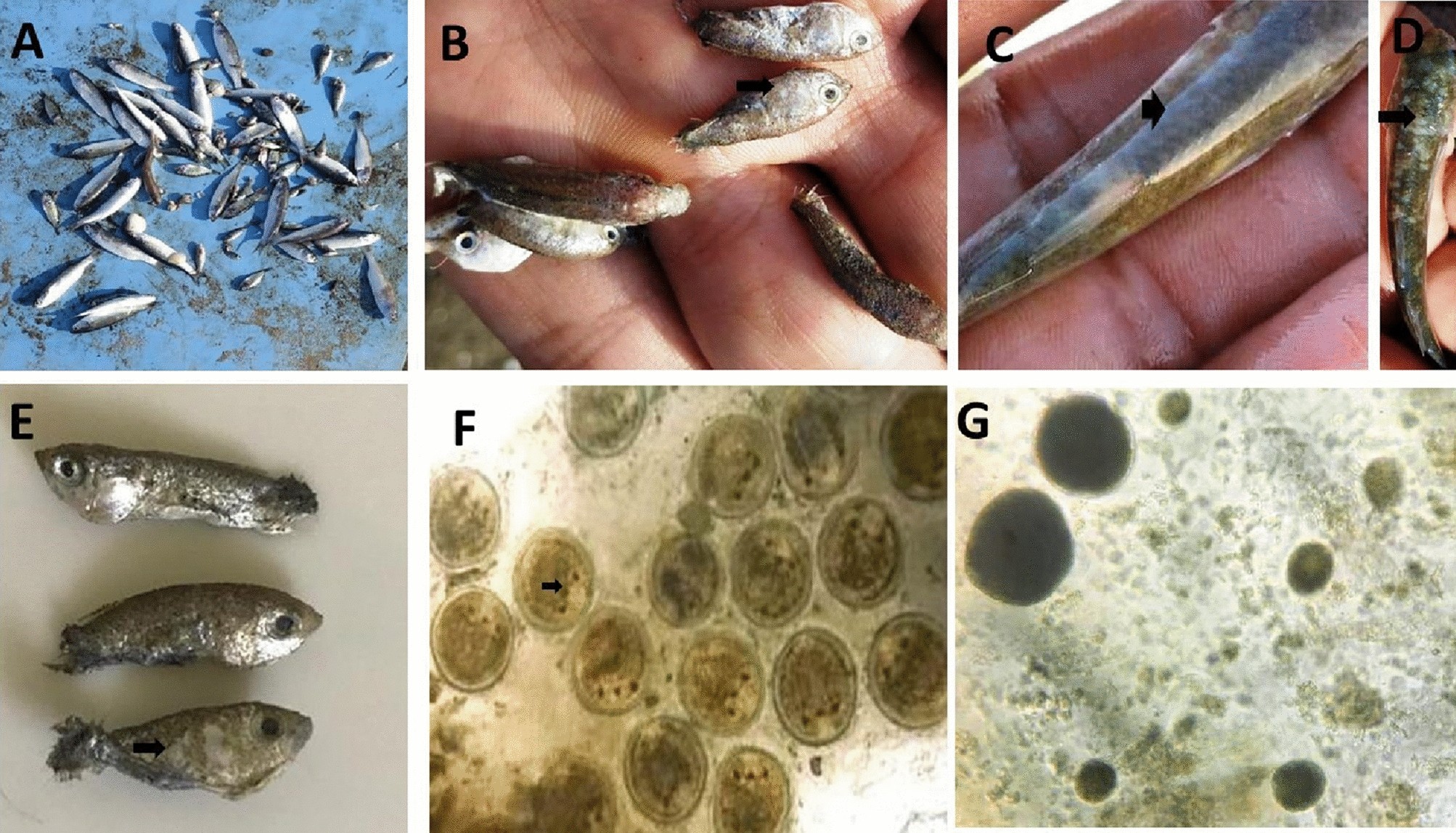This image set consists of seven images arranged in a grid, with four on the top row and three on the bottom row. Image A, located in the top left, shows a blue background covered with many small fish, resembling sardines or minnows. Image B portrays tiny fish, about an inch in size, swimming close to or eating from someone's hand. Image C features a close-up of a fish in someone's hand with a distinct black arrow pointing to its skin. The fourth image in the top row, labeled D, is partially visible with only a portion of a fish's tail observable. In the bottom row, Image E showcases three small, silver fish stacked on top of each other. Finally, Images F and G depict what appears to be microscopic views of fish eggs. Image F contains clear eggs with visible developing fish, while Image G shows darker, opaque eggs.